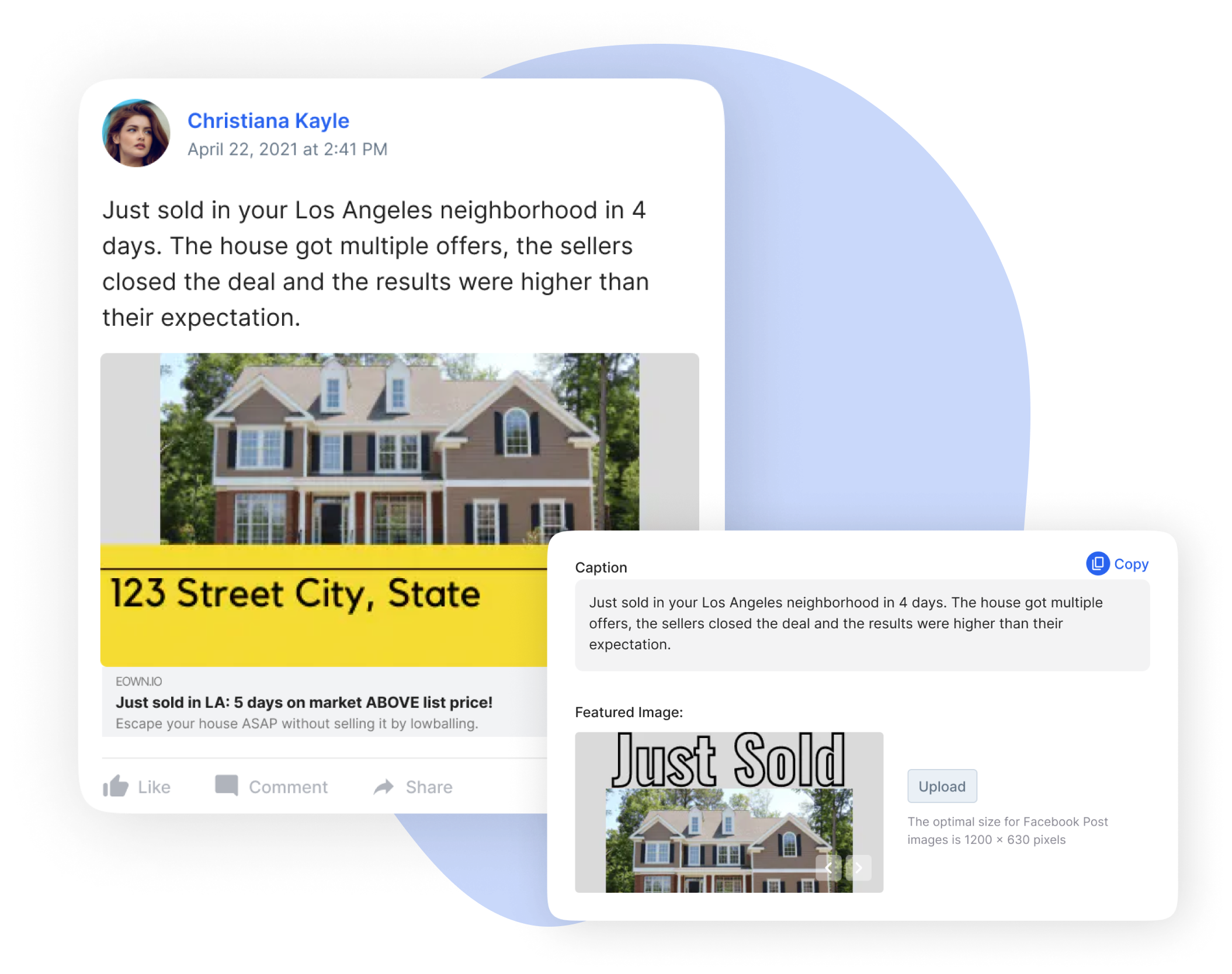**Detailed Image Caption:**

The screen capture showcases a detailed overlay of two images. In the background, a large light blue circle serves as a backdrop. The first image prominently displays a real estate advertisement featuring Christina Pale, noted in blue text. Alongside her name is a photograph of a brunette woman looking off to the side. Below her picture, the date "April 22, 2021, at 2:41 PM" is mentioned in gray text. Additional black text describes a successful sale, stating "Just sold in your Los Angeles neighborhood in four days. The house received multiple offers. The sellers closed the deal, and the results exceeded their expectations."

Beside the narrative of the sale, the image depicts a brown house with black shutters, white-framed windows, surrounded by green trees under a blue sky. A gold banner across the image reads in black text, "123 Street, City, State." Further, it notes "Just sold in LA, five days on market, above list price. Escape your house ASAP without selling it by low balling," in black and gray text.

Overlaying the bottom corner of the first image is a second image featuring another representation of the same real estate listing. This includes a white box with black text reading "Caption" and another gray speech bubble with repeating text from the original image: "Just sold in your Los Angeles neighborhood in four days. The house got multiple offers. The sellers closed this deal, and the results were higher than their expectations." A blue element labeled "Copy" appears next to an icon of stacked white papers. Below, text underscores the optimal image size for Facebook posts, indicated as "1200 by 630 pixels." Additional interactive elements include icons labeled "Like" with a thumbs up, "Comment" with a speech bubble, and "Share" with an arrow.

Prominent letters "Featured Image" and "Just Sold," outlined in black, are displayed above the repetitive image of the tan house with black shutters and white windows. A gray box labeled "Upload" concludes the information on this screen capture.